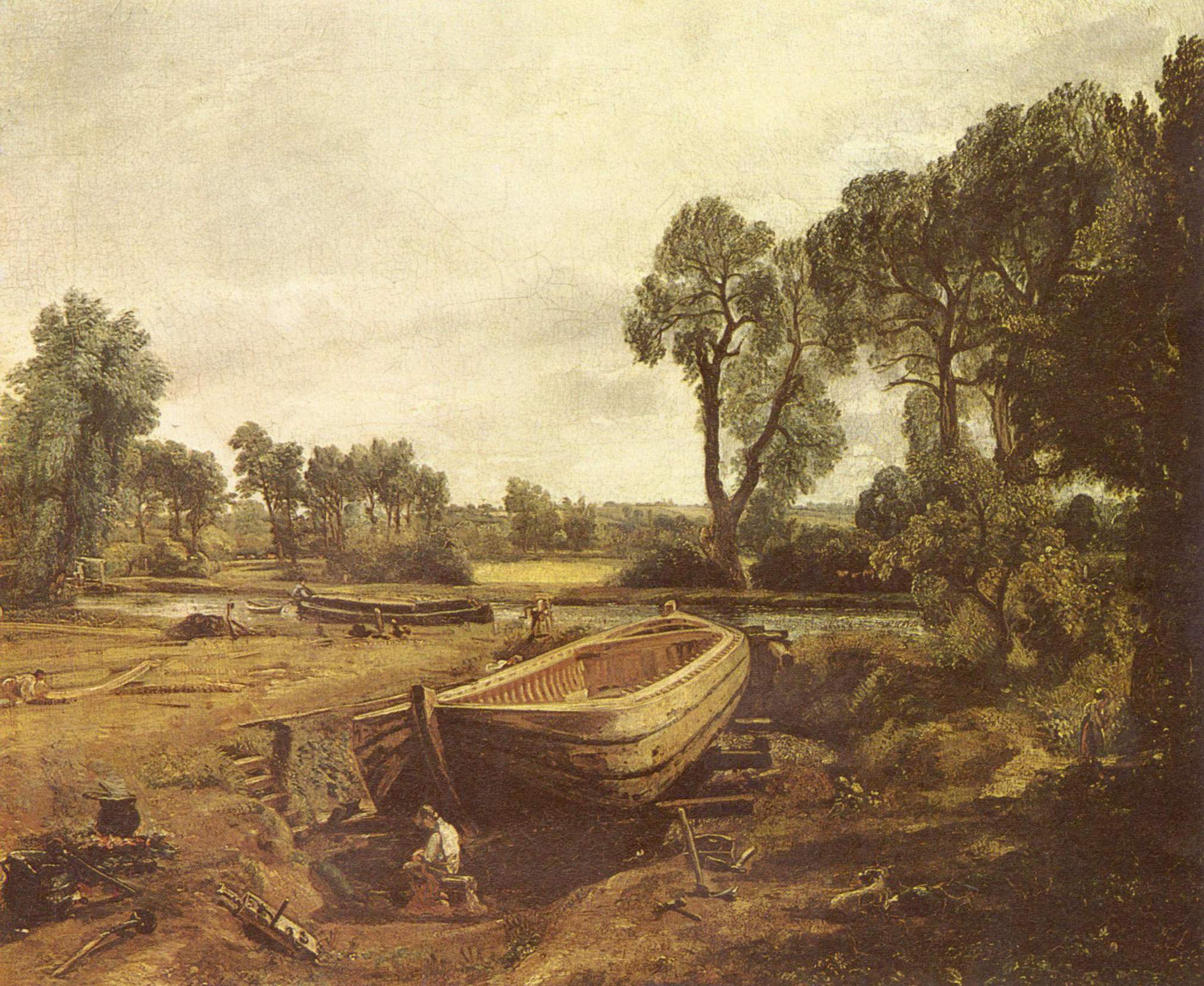This painting showcases a tranquil, outdoor scene centered around boat-building activity. At the forefront, there is an unfinished wooden boat, carved out but lacking paint or finish, resting on what appear to be railroad ties. Directly in front of the boat, a woman or possibly a young man sits contemplatively on what looks like a tree stump, surrounded by scattered tools. The ground around them is significantly dug out, with several steps leading down into the excavation, suggesting ongoing construction. Nearby, a dog lies on the ground, looking towards the woman and the boat.

To the right, another person is depicted, and off in the background, several distant figures can be seen, emphasizing a bustling yet serene atmosphere. A slightly darker boat floats on a central body of water, akin to a river, with another small boat being towed towards the shore. The middle of the image features this waterway, flanked by trees that hint at a springtime environment with their green leaves. 

The sky is overcast, casting a mix of light and shadows across the scene, with green grass and scattered rocks enhancing the natural setting. The absence of text or any artist’s signature suggests this piece might be unfinished. The overall color palette includes shades of gray, brown, and green, contributing to the earthy and calm ambiance of this nostalgic and industrious vignette.